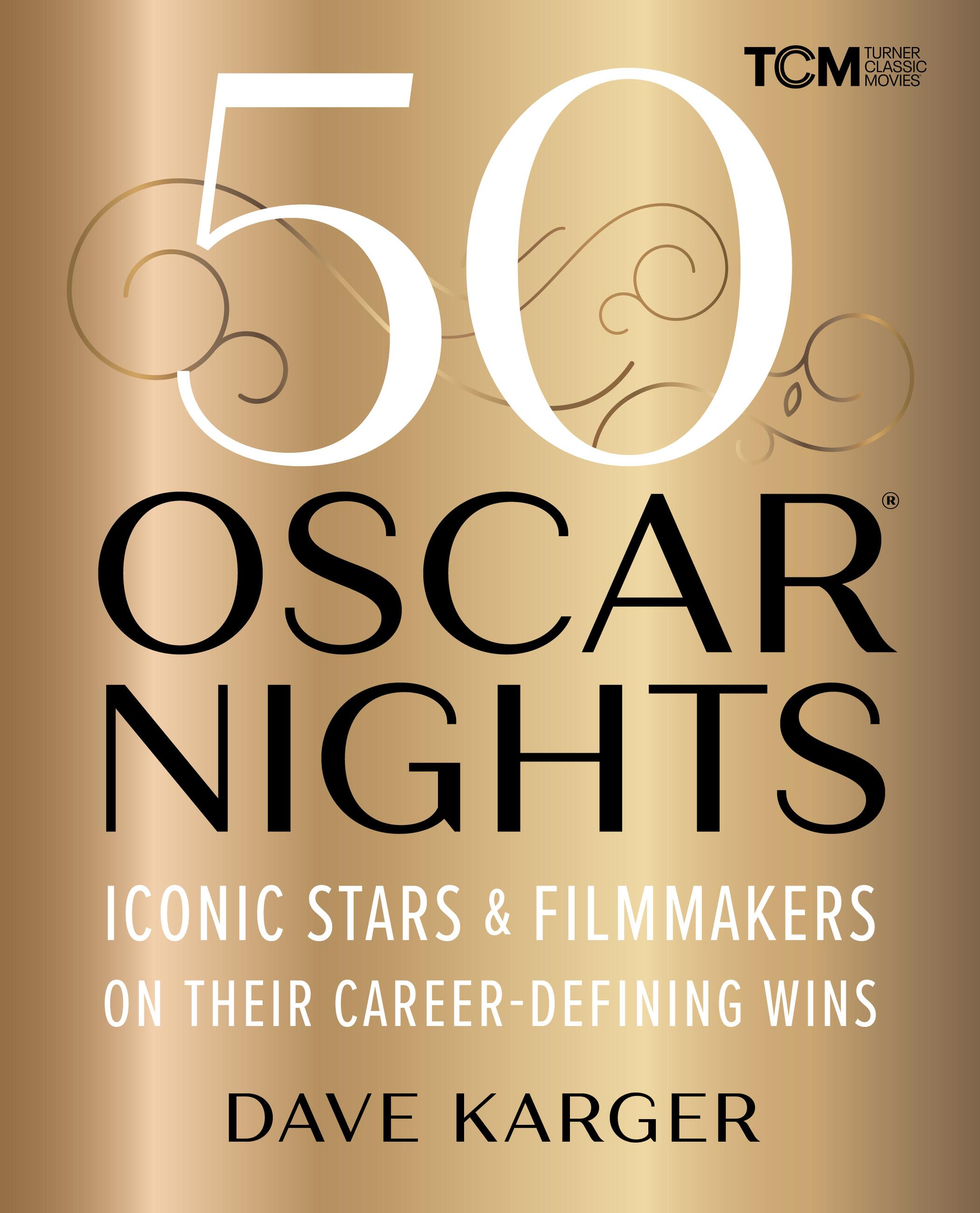The cover of this book is vertically rectangular with a gold-toned background that features varying shades, giving it a curtain-like appearance. In the upper right-hand corner, in black lettering, is the "TCM Turner Classic Movies" logo. Dominating the top center of the cover, in large white numerals, is the number "50," adorned with intricate gold swirly designs. Central to the cover, in bold black capital letters, is the title "OSCAR NIGHTS," with the subtitle "Iconic Stars and Filmmakers on Their Career Defining Wins" in white lettering underneath. At the bottom, the author's name, "DAVE CARGER," is prominently displayed in black capital letters.